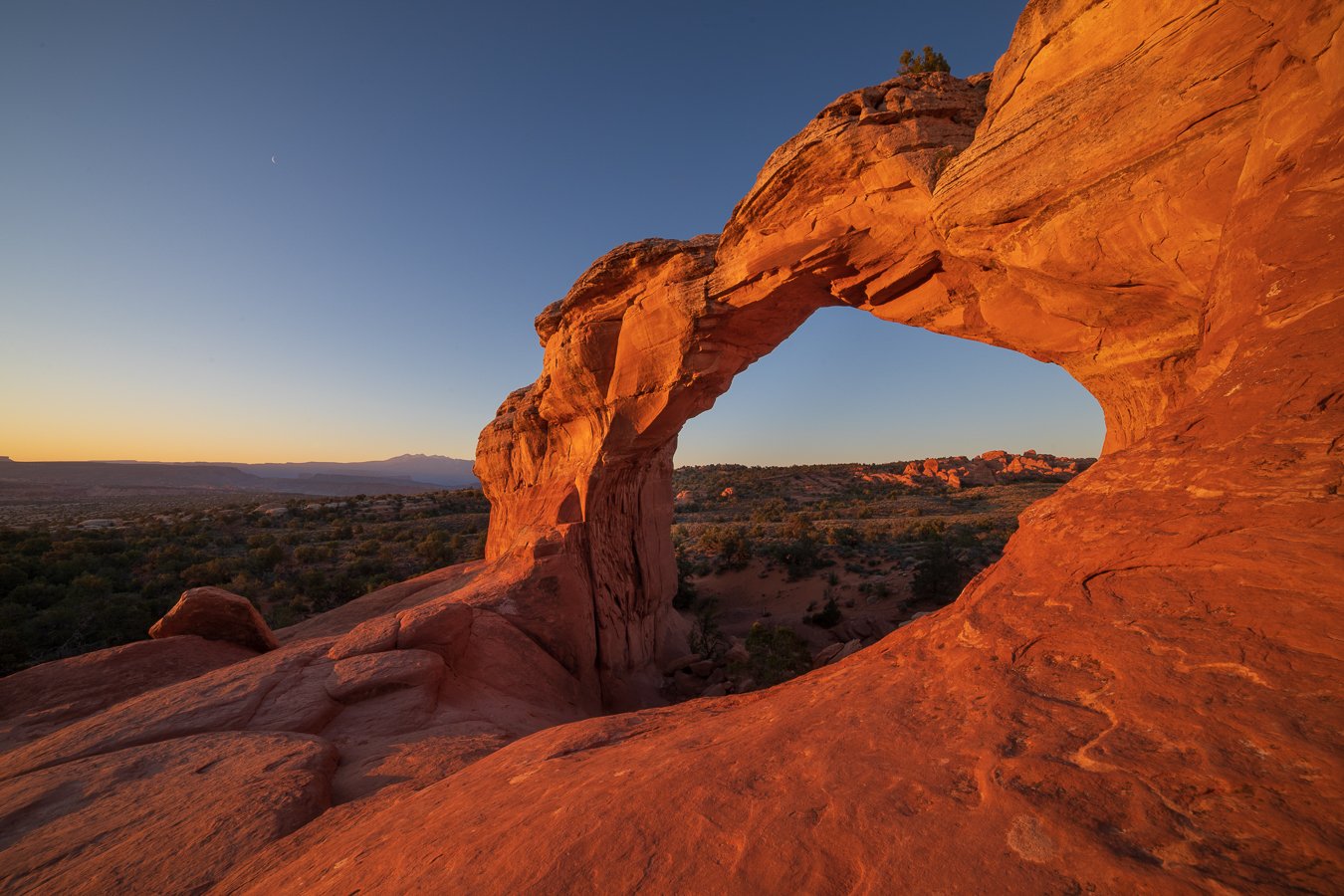The image captures a striking rust-brown and red rock formation, characteristic of the landscapes found in places like Utah or Wyoming, possibly Red Rock Canyon. The main feature is a natural rock archway that spans from the bottom left corner to the top right corner, creating a circular opening. Through this arch, one can gaze upon a distant horizon, where dark, silhouetted hills meet a clear, blue sky tinged with golden hues, suggesting that the photo was taken either at sunrise or sunset. The foreground features grassy, prairie-like lands with scattered green vegetation. The arch itself has a shadowed, dark edge at the top, adding depth and contrast to the image. Additionally, there are small patches of vegetation visible on top of the arch, enhancing the natural beauty of this iconic rock formation.